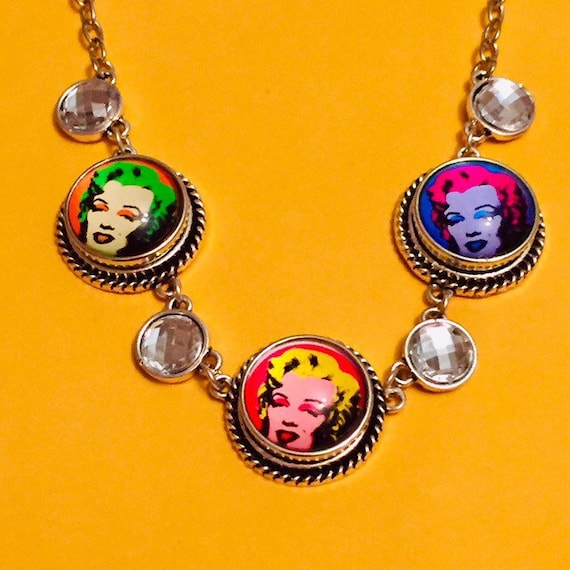This close-up photograph captures a silver necklace against a solid light orange background, hanging in a U-shape. The necklace features a series of seven round emblems arranged along a shiny metal chain. Alternating between the emblems, there are four smaller, circular rhinestones that glimmer like diamonds. Interspersed with these rhinestones are three larger circular pieces, each displaying a pop art image of Marilyn Monroe. From left to right, the first emblem showcases Marilyn with green hair, orange eyeshadow, and dark orange lipstick. The second emblem features her with blonde hair, hot pink eyeshadow, and lips framed by a pink background. The third emblem presents Marilyn with striking hot pink hair, blue eyeshadow, and matching lipstick against a blue background. The vivid contrast between the rhinestones and the colorful depictions of Marilyn Monroe creates a visually captivating piece of jewelry.